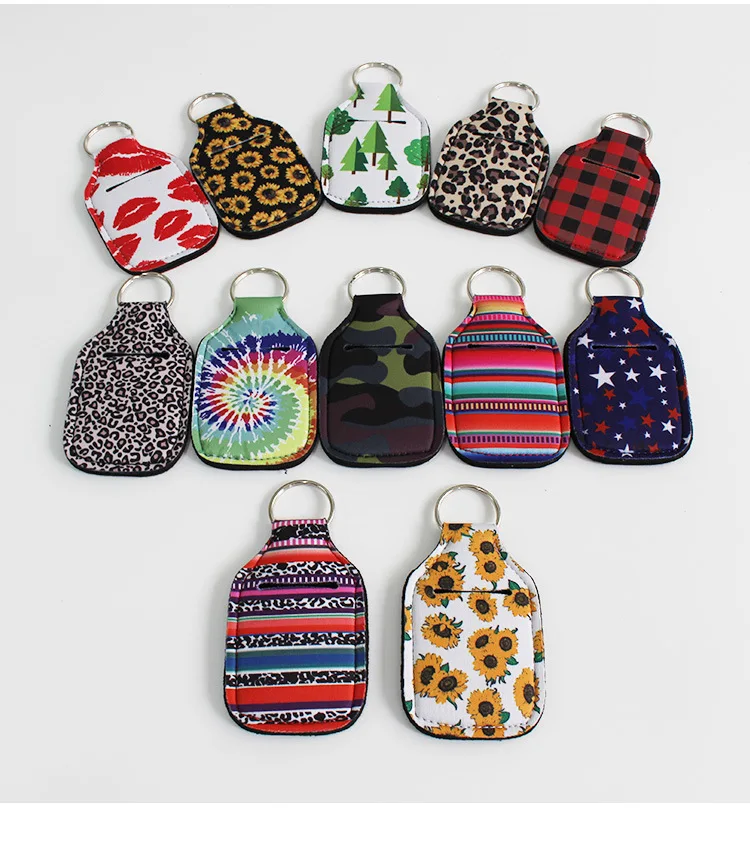The image displays a collection of 12 custom keychain holders arranged in three rows. Each keychain holder has a silver ring at the top and various unique designs and patterns on the bottle-shaped body. The top row consists of five keychain holders. The first is white with a red lips pattern, the second features black with sunflowers that have black centers, the third is adorned with green evergreen trees on a white background, the fourth has a tan base with large leopard prints, and the fifth demonstrates a classic red and black mackinaw checkered pattern.

The second row, also consisting of five keychains, continues with a varied display: the first is tan with small leopard prints, the second displays a circular snail shape with a rainbow tie-dye effect, the third is camo in shades of green, black, and purple, the fourth presents a straightforward fabric design in solid colors, and the fifth is dark blue with white, blue, and red stars.

The bottom row holds the final two keychains. The first exhibits a camo pattern, and the second is red with yellow flowers. All keychains are made of either cloth or rubber, adding distinct textures to their vibrant designs.